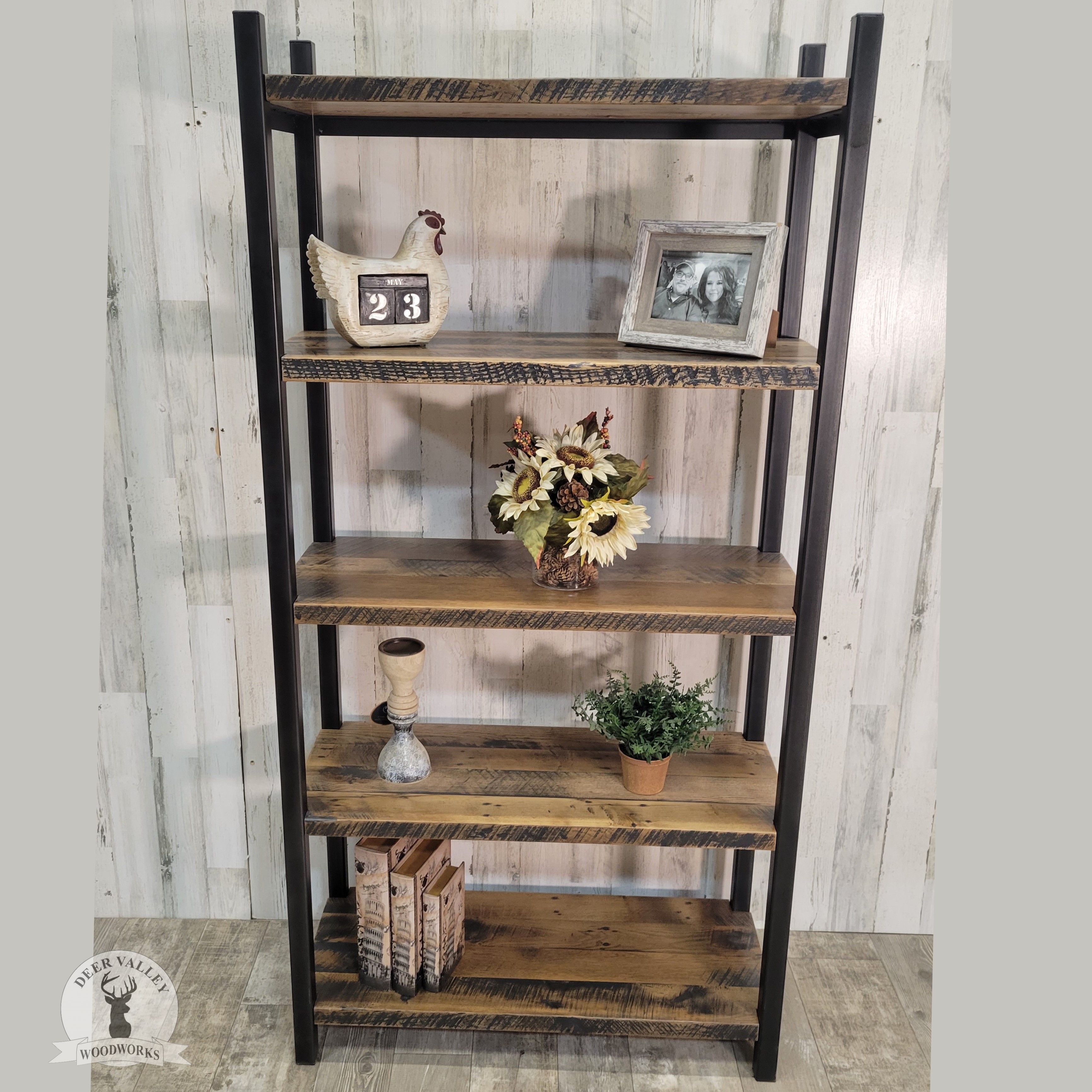The photograph features a rustic, multi-shelf wooden piece of furniture designed for displaying personal items, often found in a living room setting. The furniture appears to be weathered, giving it a vintage charm with its dark wood grain against a backdrop of a white, unevenly stained wall. There are five shelves in total.

On the top shelf, a ceramic chicken acts as a calendar, showing the date "23 May 23." To its right, a tan photo frame holds a black and white image of a man wearing a cap and a woman with voluminous hair. The second shelf below holds a vase filled with light yellow fake sunflowers, accented with some pine cones and smaller filler flowers.

The third shelf features a small green plant in a terracotta or plastic planter. Below it, on the fourth shelf, are three wooden books stacked neatly, with "Deer Valley Woodworks" etched in the bottom left corner of the furniture. The background and floor share a similar color palette, being primarily white with gray, uneven spots, complementing the overall rustic aesthetic of the display.